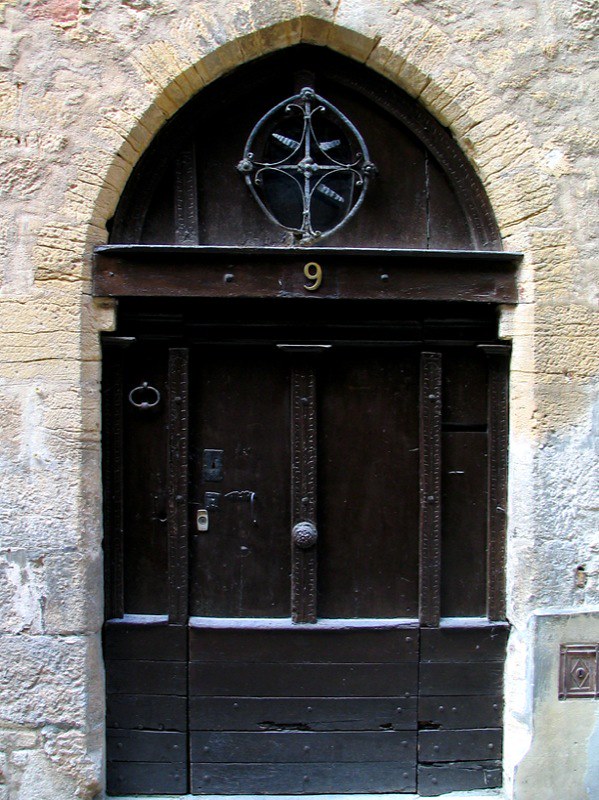This color photograph showcases a close-up view of a robust and antiquated arched doorway set within a sturdy and elaborate brick and stone wall. The wall appears predominantly whitish-gray with hints of yellow around the arch. This arched entryway leads to a heavy, dark brown wooden door, composed of meticulously arranged blocks of wood at the bottom, vertical bars in the middle, and horizontal boards at the base. Positioned at the center of the door is a keyhole, a handle, and a knocker. Above, a gold number 9 is prominently displayed near the top of the door. Encompassing the arch is a circle featuring an intricate metal design that includes interconnected spirals or protrusions, suggesting a cross-like, ornate pattern. This doorway encapsulates the historic charm and solid workmanship typical of old buildings, possibly a church or a similarly venerable structure.